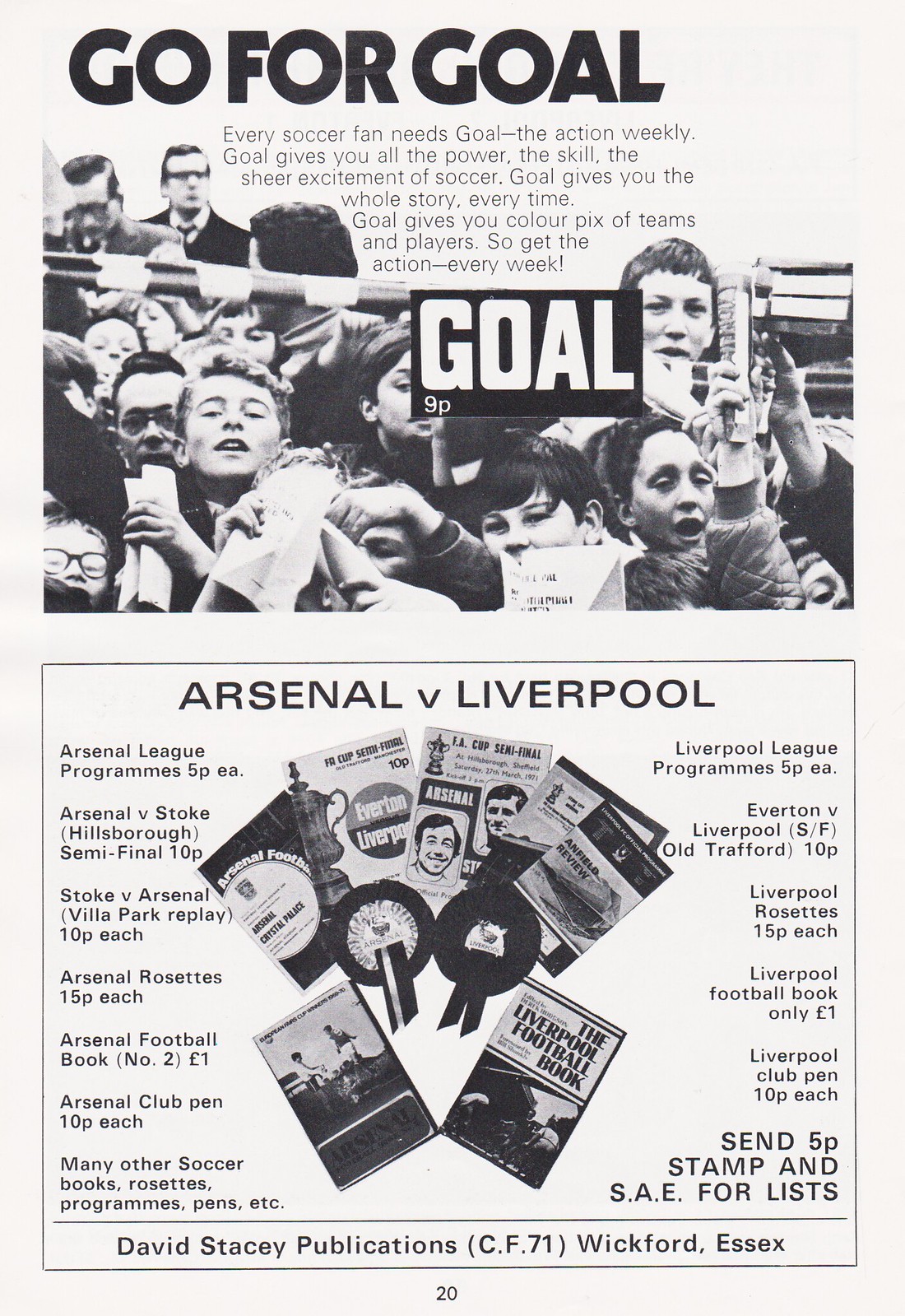**Caption:**

This monochromatic magazine cover, titled "Go for Gold," is a treasure trove for soccer enthusiasts. The top of the page boldly declares, "Every soccer fan needs Gold. The Action Weekly Gold gives you all the power, the skills, and the sheer excitement of soccer." Beneath this tagline, readers are promised comprehensive stories and vibrant color pictures of teams and players, though the current issue features black and white imagery. Dominating the page is a crowd of jubilant fans, possibly in a stadium, beaming at the camera.

Below the photograph, there's an advertisement for an Arsenal v. Liverpool match, with additional references to a variety of available football programs surrounding the central image. These programs are published by David Stacey Publications, CF71 Wickford Essex. The promotional material also lists the costs and details for ordering the magazines. Toward the bottom is the reference "Page 20," indicating its place within the greater publication.